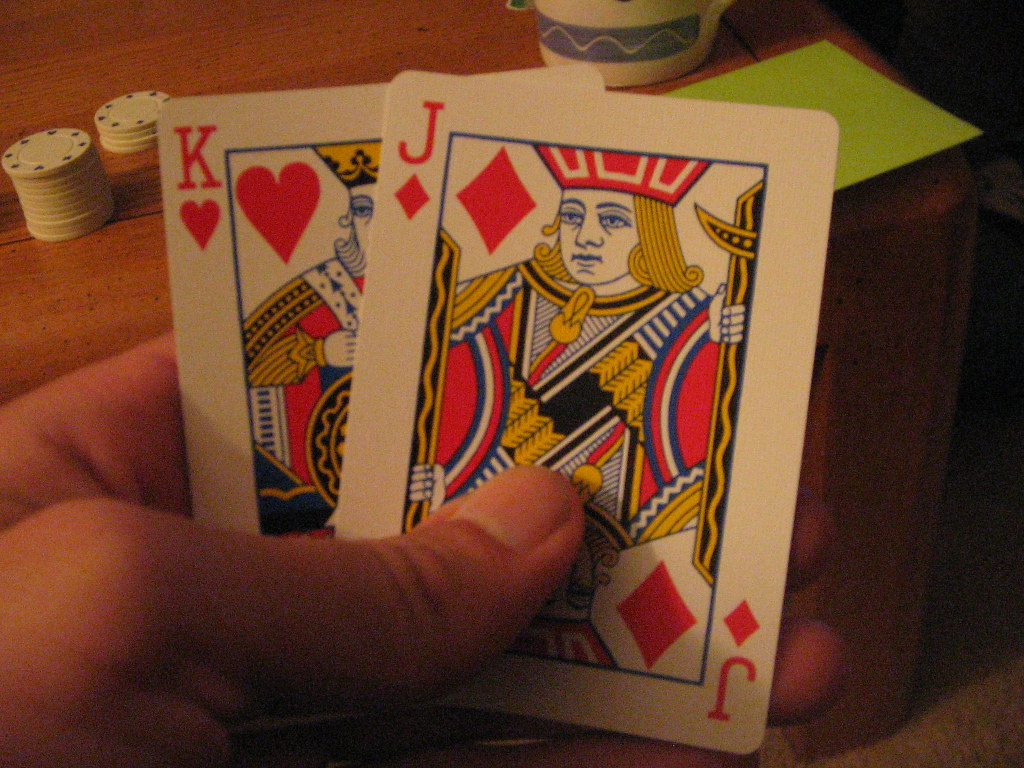In this vivid photograph, situated on the left side, a human hand delicately holds two playing cards between the forefinger and thumb. The card on the right is the Jack of Diamonds, distinguished by its intricate design featuring gold-yellow hair, a red and blue uniform with white and blue accents, and an object in his hands. The card on the left is the King of Hearts, partially obscured by the Jack. However, the visible details showcase a regal golden crown and a uniform adorned with gold, red, blue, and touches of black.

In the background, a poker game is in progress. To the right of the hand, a neat stack of approximately ten white poker chips is positioned, signifying potential winnings or bets. Just beyond this, another smaller stack of four white chips can be seen, possibly part of a recent play. A green piece of paper lies on the playing surface, likely serving as a scoresheet or note of game points.

The entire scene captures the intensity and detail of a moment in a poker game, with the elaborately decorated cards and carefully stacked chips adding a rich texture to the image.